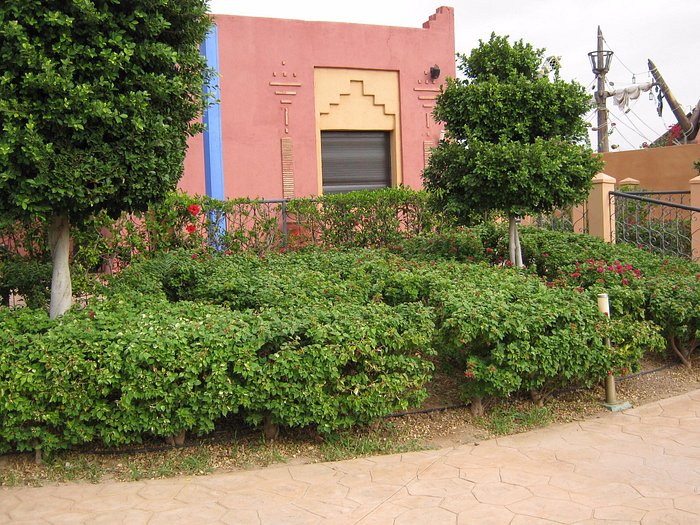The image depicts a one-story, salmon-colored building with a flat roof, accented by a gold-painted window. Positioned behind two lush green trees and various shrubs, the building features a blue light pole to its left. The entrance of the building has a distinct design with a yellow top and dark brown bottom. In front, there is a weathered metal fence adorned with thriving plants and vines. The scene is set on a cobblestone walkway and further enhanced by a basket-shaped structure atop a pole. In the distant background, partially obscured by a concrete fence, the mast of an old-time sailship with hanging sails and a crow's nest can be seen, adding a touch of historical intrigue to the setting. The overall scene combines elements of greenery, historical maritime aesthetics, and quaint architectural details.